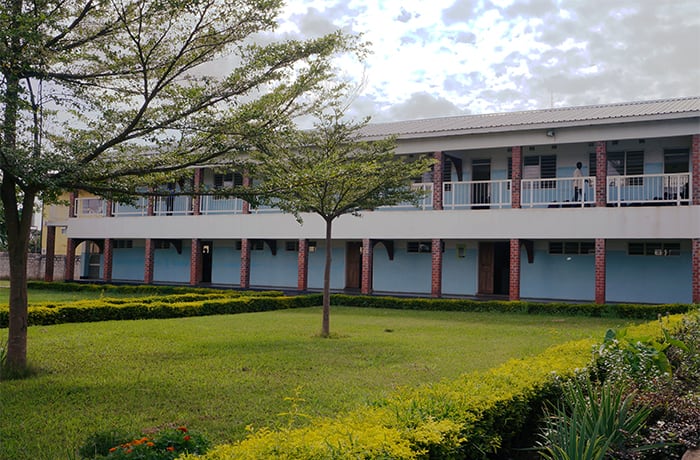This image captures a well-maintained, two-story building that appears to be a hotel or residential apartment. The building is painted light blue and features a tin roof. Its second story is distinguished by white railings that span between brick support columns, while the ground floor also boasts brick columns but lacks fencing. A neatly manicured landscape garden adorns the front of the building, characterized by a vibrant green lawn bordered by hedges. Two trees occupy the center of the garden; one is fully grown, while the other is still maturing. Additional shrubbery is located in the far right-hand corner. The background showcases a blue sky with some scattered gray, puffy clouds. A person can be seen walking along the second-floor hallway, though their details are indistinct. The overall scene is rich with colors, including shades of green, blue, gray, brown, white, yellow, and pink, creating a picturesque outdoor setting.